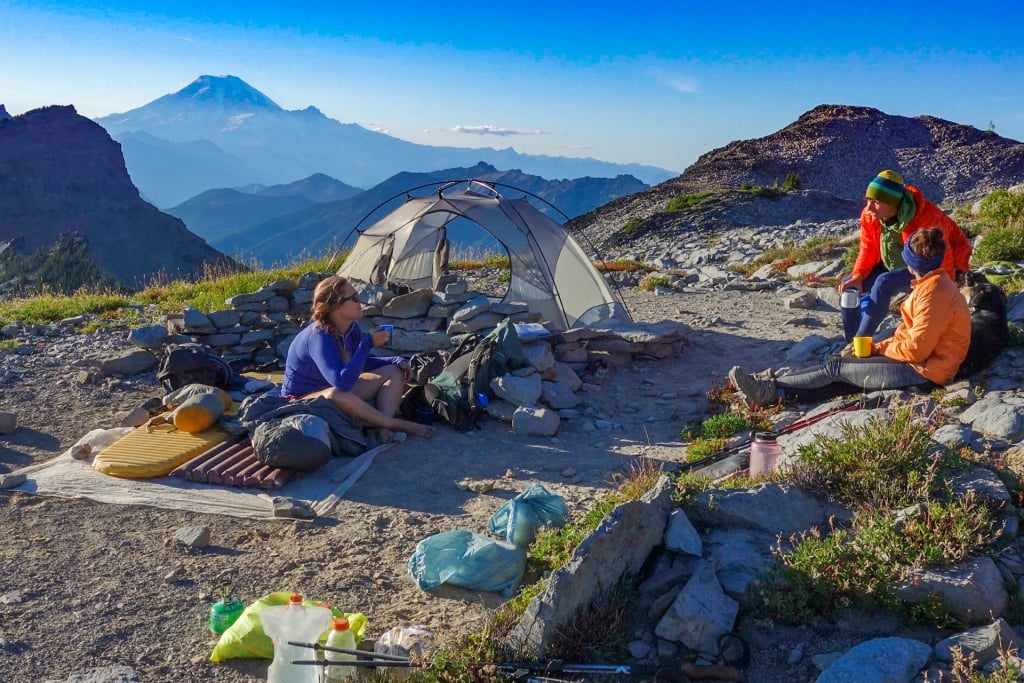This image captures a serene camping scene atop a desolate, rocky mountain range under a clear blue sky. Three people are featured, set against a backdrop of cascading mountain ranges that fade from dark to light blue in the distance. The foreground is a dusty, dirt surface dotted with greenery and scattered camping supplies, including Gatorade bottles, air mattresses, and bags.

Positioned slightly to the left, a woman wearing a blue long-sleeve shirt and shorts sits comfortably on the ground, holding a blue cup of coffee. She's framed by a small, gray dome tent surrounded by a protective rock wall. To the right, a man in a vibrant orange ski jacket and yellow-blue-green ski cap converses with a woman in a lighter orange jacket, gray hiking pants, and boots. Both are seated on rocks and appear engrossed in their morning dialogue, each with a cup of coffee in hand.

Despite the dry, barren landscape devoid of trees and teeming with rocks, the scene glows under the bright morning sun. Shadows stretch lightly across the ground, heightening the sense of tranquility and picturesque beauty in this mountain-top camping experience. The overall atmosphere is one of calm, happiness, and connection, as the campers share a peaceful moment, basking in the splendor of their natural surroundings.